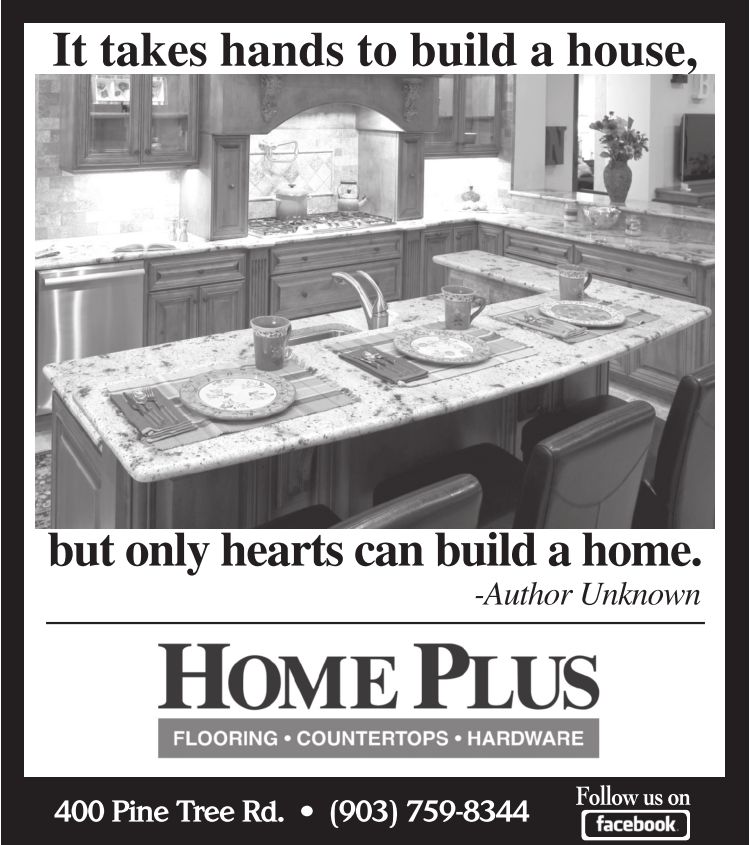This black-and-white advertisement for Home Plus features a stylish kitchen framed by a heavy black border. The kitchen showcases a marble countertop island with three place settings and chairs, facing a sink across the counter. In the background, nine pine cabinets, some with glass fronts, a stove, and additional cabinetry complete the scene. The ad emphasizes its message at the top with "It takes hands to build a house," followed by "but only hearts can build a home" at the bottom, credited to an unknown author. Beneath this quotation, a fine black line separates it from the large, capitalized text "HOME PLUS," accompanied by a gray rectangle highlighting "Flooring. Countertops. Hardware." The footer of the ad provides the address, "400 Pine Tree Road," and contact details, "(903) 759-8344." Additionally, the bottom-right corner encourages viewers to "Follow us on Facebook."